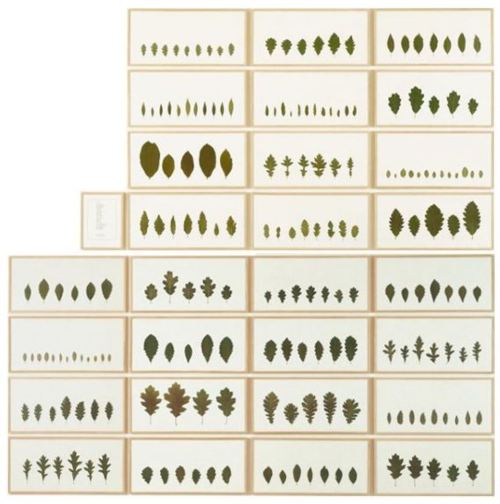The image depicts a detailed chart consisting of a rectangular grid featuring a series of smaller rectangles arranged in four columns. The leftmost column consists of only four rows, including a partial row at the top, whereas the other three columns contain eight rows each. The chart showcases a variety of leaves displayed within these rectangles, which are stacked on top of each other. There are three primary styles of leaves: one resembling small clamshell shapes, another with more vertical, oval-shaped leaves, and a third displaying larger leaves with many intricate cuts, giving them a multi-leaf appearance. The leaves range in color from dark green to olive green, suggesting different stages of growth. In the middle-left section of the grid, there's one small rectangle that contains an unidentifiable object. The overall layout lacks a discernible pattern, emphasizing the diverse nature of the leaf samples included.